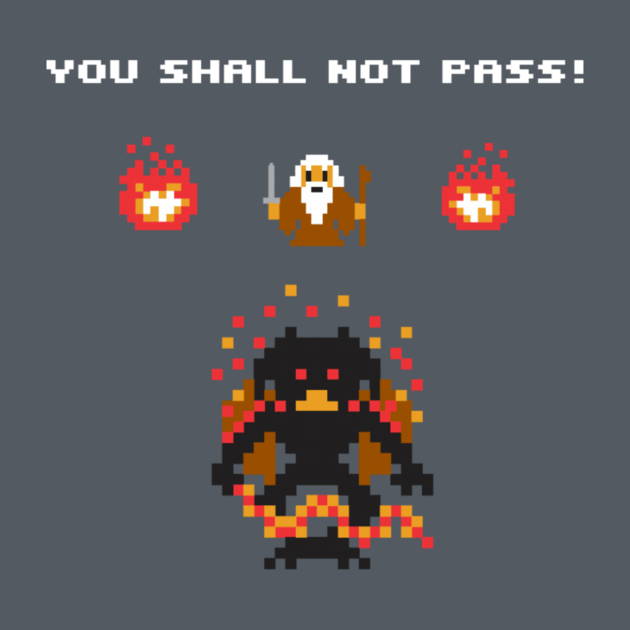The image, taken from a retro-style video game, features a solid dark gray square background. Centered at the top in all-cap white letters, it proclaims, "YOU SHALL NOT PASS!" Below the text, three distinct pixelated elements dominate the upper part of the image. 

In the center, there's a bearded man dressed in a brown robe, wielding a gray sword in his right hand and a brown staff or axe in his left hand. His eyes are black, and his long white hair and beard give him a wizard-like appearance, reminiscent of Gandalf. Flanking him on both sides are small, pixelated flames. Each flame has a white and brown center encircled by a round red border with little red dots floating upwards, adding dynamic energy to the scene.

Beneath the robed figure is a larger black creature with prominent red eyes and a brown mouth. This menacing figure has ears that hang down and appears poised to attack, arms outstretched to the sides. Surrounding it are various colored squares, primarily red, orange, brown, and yellow, enhancing the fiery, chaotic atmosphere.